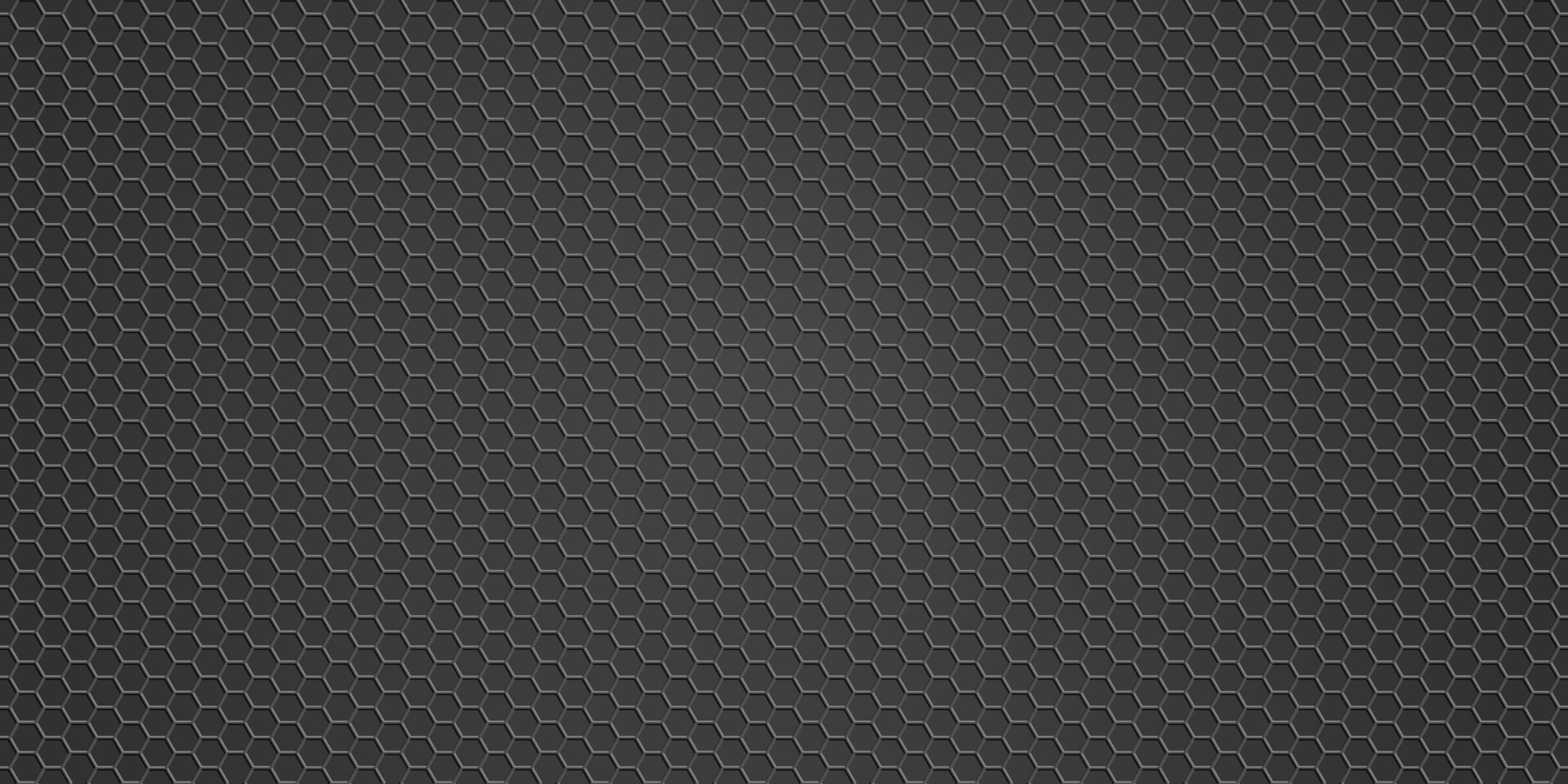The image is a color illustration in landscape orientation featuring a dark gray, almost black background with a distinct honeycomb or hexagonal pattern. This pattern consists of thousands of interconnected, lightly stroked hexagons in a lighter gray or white color, resembling a net or beehive design. The hexagons are organized in vertical columns, creating a mesh-like effect that extends across the entire image from left to right and top to bottom. Each row vertically contains approximately 15 to 20 hexagons. The overall image has a narrow, wide format, emphasizing the intricate, repeating pattern of the hexagons against the deep gray background.